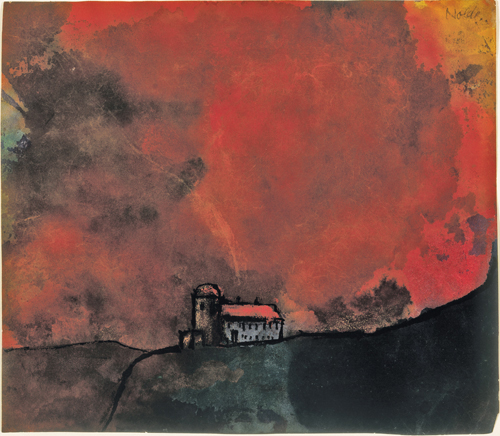This image is a detailed painting depicting a small, modern farmhouse situated in the center bottom of the canvas. The farmhouse, featuring a white facade with a red gabled roof, stands prominently atop a hill. Accompanying the farmhouse to its left is a classic silo with a dark gray body and a red domed top. The painting employs various shades of black, dark red, and mustard yellow blended together to create a dramatic sky that suggests either a sunset or possibly a wildfire in the background. The bottom part of the hill where the farmhouse rests is divided into two distinct areas: a solid black shadowed region occupies the bottom right corner, while a splotchy gray section spreads across the left and middle portions of the hill. These colors might have been applied in a watercolor-like fashion, enhancing the fluid, dynamic quality of the landscape. Additionally, a small, dome-topped building is visible to the left of the silo, adding to the rustic charm of the scene. The artist’s possible signature appears near the top right corner of the painting, adding a personal touch to this evocative artwork.